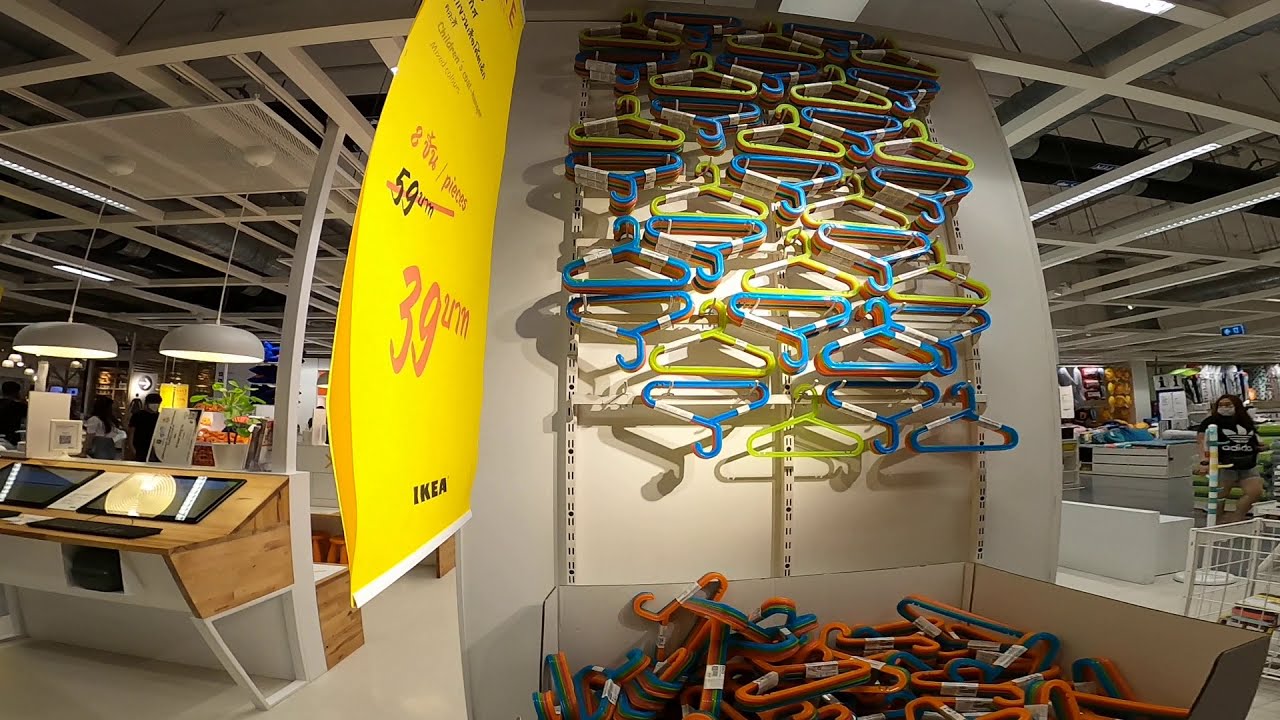This photograph captures a section of an IKEA store showcasing a colorful array of clothing hangers. The hangers, available in vibrant hues of red, blue, yellow, and orange, are meticulously arranged on a vertical wall display, some even hanging upside down. Below the wall display, there's a bin filled with more hangers, haphazardly stacked in various colors. Positioned to the left of the display, a prominent yellow and white IKEA sign provides pricing and date information, clearly indicating the store's characteristic look and atmosphere. Surrounding this focal area, additional IKEA product displays can be observed, including desks to the left and a fenced-off bin area to the right. In the background, various light fixtures illuminate the scene, and several shoppers, including a woman wearing a face mask, move through other parts of the store. Despite some areas being less distinct, the overall image conveys the bustling yet organized environment typical of IKEA.